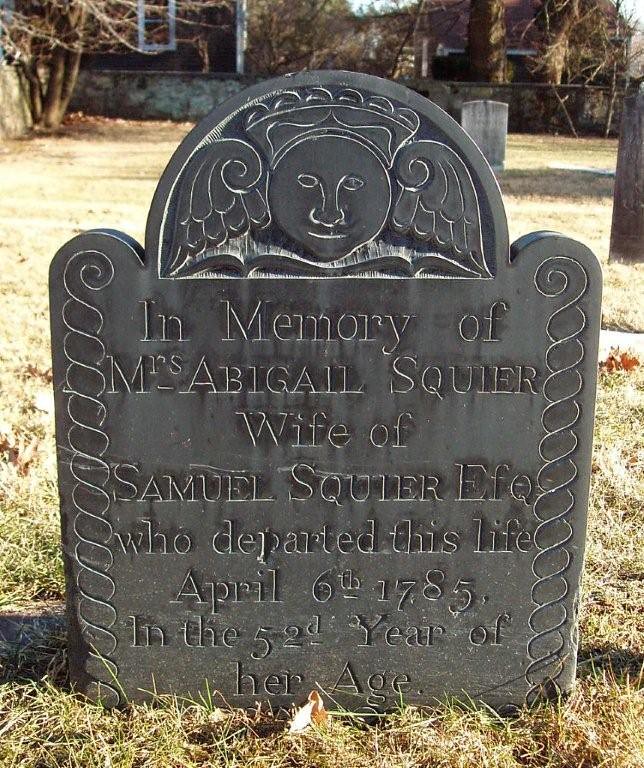The image depicts a detailed gravestone standing prominently in the center of a bleak, barren landscape. The gravestone, made of dark, silvered granite, features an intricate design: a face adorned with a crown and flanked by angelic wings, set atop a book-like structure. The sides are embellished with swirling, interconnecting lines resembling a cane design. The inscription reads: "In memory of Mrs. Abigail Squire, wife of Samuel Squire Esq., who departed this life April 6, 1785, in the 52nd year of her age." The background reveals an expanse of yellowed, almost burned grass, typical of a dry or winter season. There are a few other gravestones dispersed across the scene, along with a building or structure and a window in the far distance. The presence of leafless trees and possibly a wooden fence can also be observed, creating a somber, yet clear and well-focused composition that emphasizes the gravestone as the central subject of the photograph.